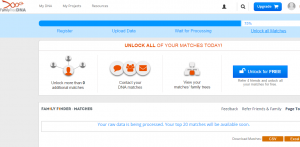The image is a low-resolution screenshot of a website's homepage, appearing cropped and zoomed in, which affects the clarity and legibility of the details. The homepage utilizes a primary color scheme of white, orange, and blue.

In the top-left corner, there is a logo featuring a red double helix design, suggesting a twisty pattern. Adjacent to the logo are three navigation tabs. On the top-right corner, there's an "Upgrade" option, followed by a shopping cart icon. To the right of these elements, there’s a search button which likely expands into a search bar upon interaction. Flanking the search button and the "Upgrade" button are two profile picture symbols.

Directly below this header section is a blue bar that could be a loading or progress indicator, accompanied by three clickable text tabs underneath it.

The central message on the page reads, "Unlock all of your matches today." The main content area is divided into four sections, three of which are illustrated with orange and white graphics. The section on the right features a blue button labeled "Unlock for Free," accompanied by an unlock symbol. 

Further down, the website presents additional content with text that is mostly illegible in this low-resolution screenshot. However, at the bottom-right corner, there are two more orange buttons, their text indistinguishable.

Overall, the screenshot attempts to capture the functional layout and design elements of the homepage, albeit with limited clarity.